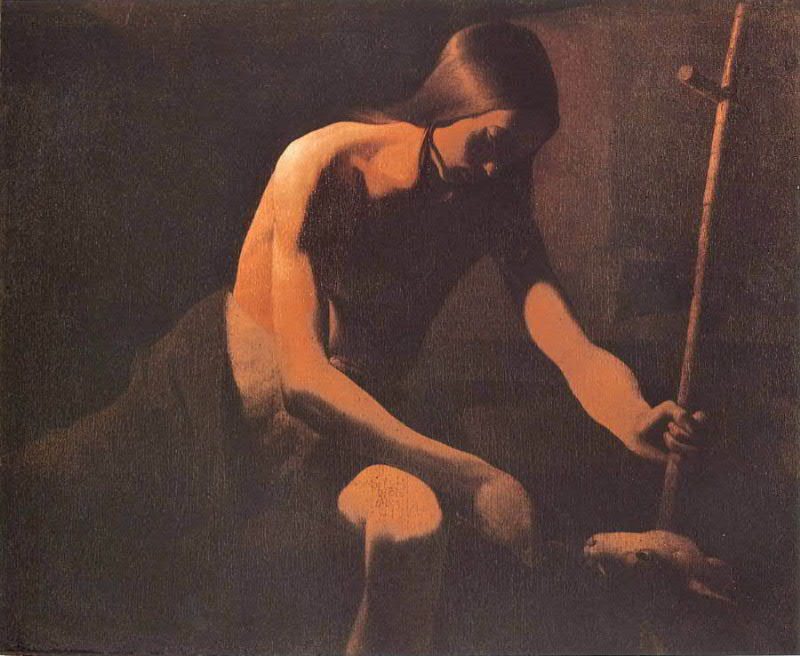In this deeply shadowed, almost monochromatic painting, the central figure—a shirtless man with long black hair, likely of Native American origin—sits or kneels in a dimly lit room, possibly a cave. The room is dark with an orangish, reddish glow emanating from a light source behind him on the left, casting an enigmatic ambiance. Draped in a loosely tied brown blanket around his waist, the man’s right arm holds a stick resembling a cross, which appears to pierce the head of an animal, likely a lamb, resting on a wooden table in front of him. His left hand offers food to the lamb, which in turn sniffs at it cautiously, its ears laid back. The background is obscured, with details shrouded in darkness, adding to the painting’s mysterious and contemplative mood.